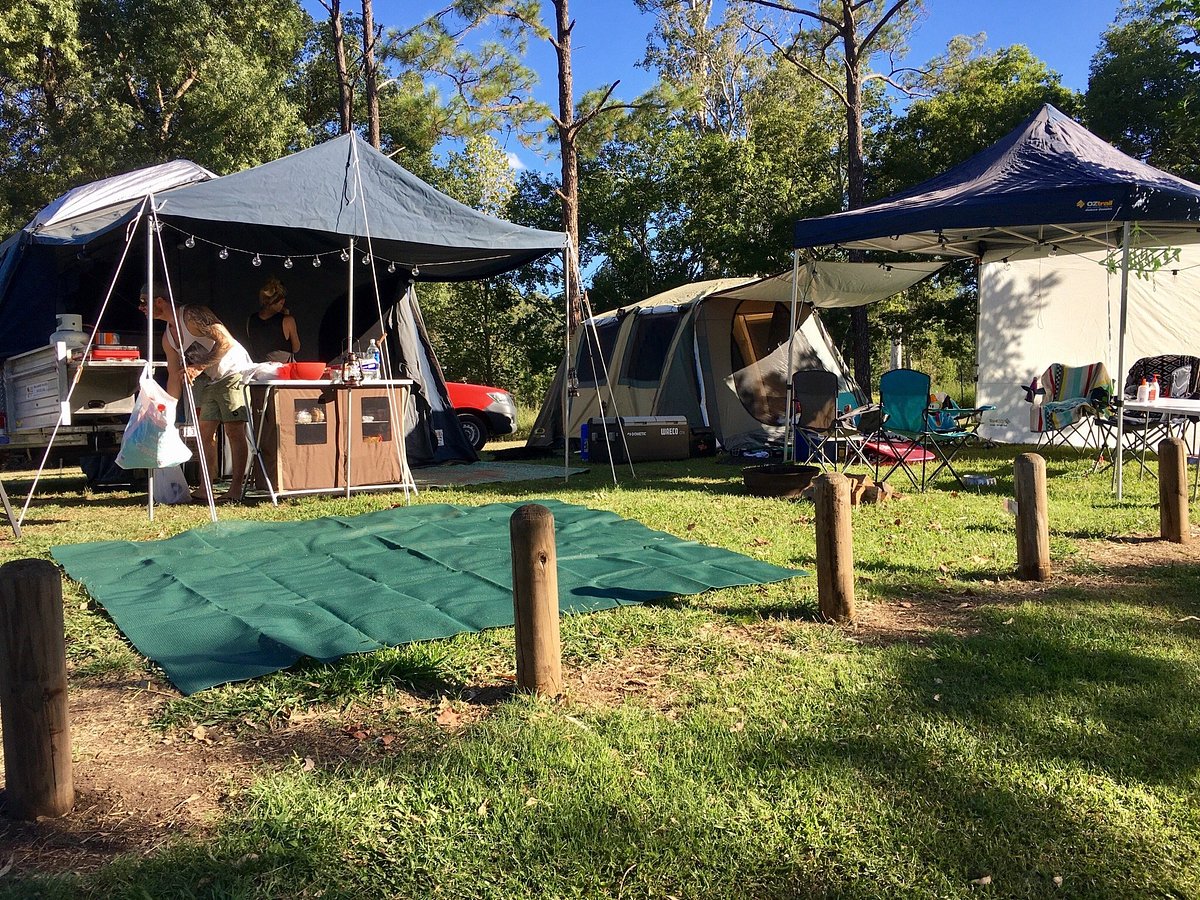This photograph captures a bustling campsite set on a grassy terrain. The site is demarcated by wooden posts, ensuring separation from neighboring campsites and protecting tents from vehicular intrusion. Central to the scene is a gray tent pad that shields the tent from ground moisture and condensation. Adjacent to this is a prominent setup of canopy tents providing shelter and space for varied campsite activities.

Under one canopy, a table and four folding chairs are arranged for comfort. Nearby, another elaborate canopy functions as a makeshift outdoor kitchen, complete with a cook stove, various kitchen supplies, and a person — possibly a man — engaged in cooking. This comprehensive setup includes a stand covered with brown fabric, over which a white tarp and a green tarp have been strategically placed for additional protection. Notably, the structure features orange bows and a hanging plastic bag, indicating practical storage.

Between the canopies stands an enclosed tent designed for sleeping, with a cooler positioned at its entrance. The whole scene is flanked by a red pickup truck, hinting at the campers’ mode of arrival. In the background, other tents, a car, and lush trees under a blue sky complete the picturesque and lively outdoor setting.